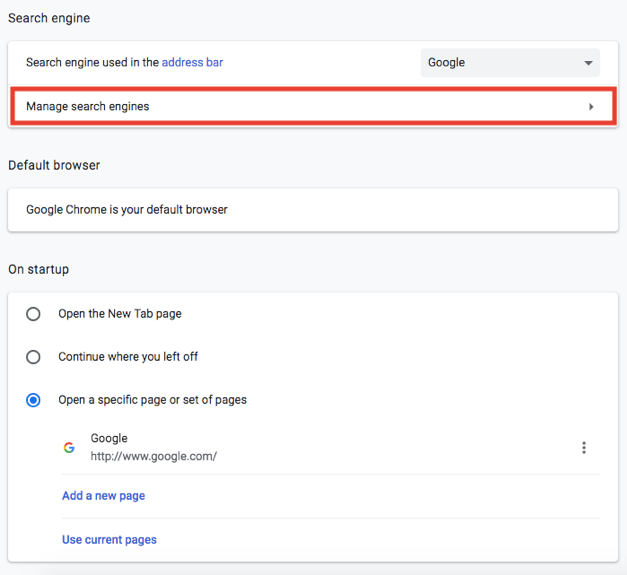[Detailed Caption]

The image features an interface with a predominantly gray background scattered with various white rectangles of different sizes. At the top of the interface, 'Search Engine' is prominently displayed in black text. Below this, a large white rectangle houses the label 'Search Engine User' and contains a blue address bar.

Just beneath this section is another white rectangle, bordered in red, featuring the text 'Manage Search Engines' in black. The term 'Default Browser' follows below this, accompanied by more white space. Further down, another white rectangle with black text declares 'Google is your default browser.'

Continuing downward, the interface shows different startup options within another white rectangle. These options, listed in black text, include: 'Open a new tab page,' 'Continue where you left off,' and 'Open a specific page or set of pages.'

Next, the familiar multi-colored 'G' logo of Google is evident, accompanied by the URL 'http://www.google.com' in black text underneath. Adjacent to this are three small black circles in a horizontal alignment. A thin gray line stretches almost the full width of the white rectangle, partitioning the section visually.

Below this line, 'Add a new page' is highlighted in blue, followed by another thin gray line. At the very bottom of the interface, 'Use current pages' is displayed in blue, signaling another interactive option.

The structured and detailed layout effectively outlines various settings and actions related to managing search engines and startup pages.